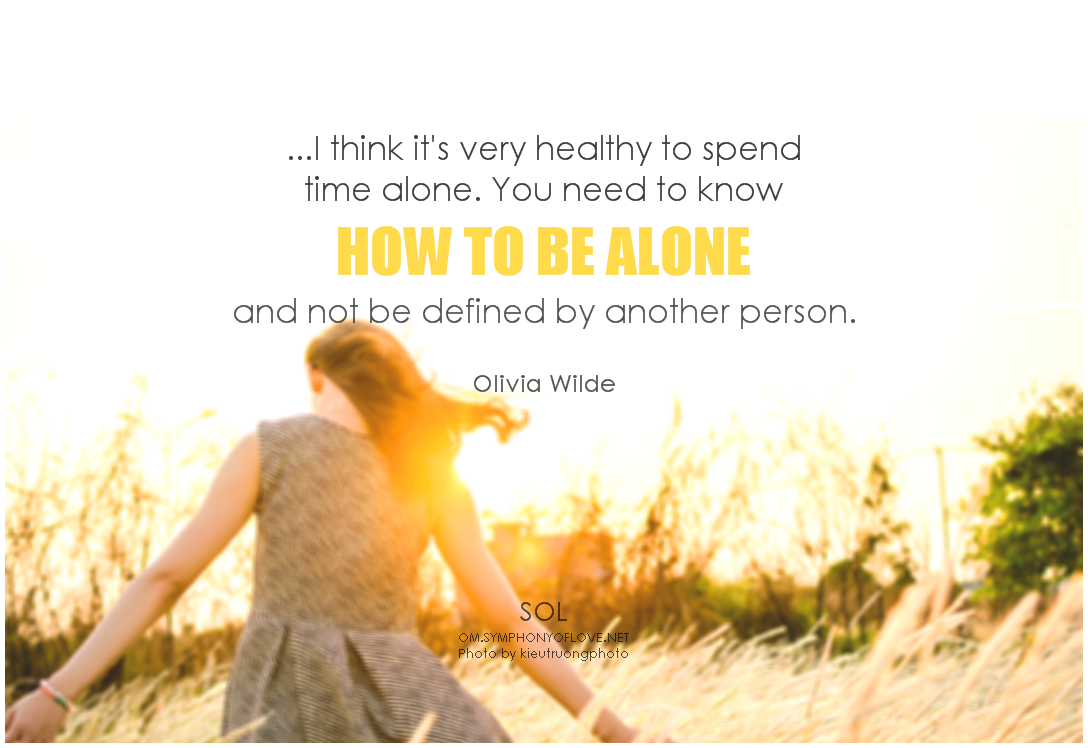The image is an inspiring advertisement featuring a famous quote by Olivia Wilde. The central feature is a photograph of a woman, with reddish-brown hair, wearing a gray dress that flows in the wind. She walks away from the camera, arms outstretched, gently touching the tall, golden wheat around her. The scene is bathed in bright sunlight, giving the image a warm, ethereal quality. In the distance, a line of green trees and a large house can be seen. 

Overlaid on the image, the text reads: "I think it's very healthy to spend time alone. You need to know how to be alone and not be defined by another person." The segment "how to be alone" is highlighted in bold, yellow text, while the rest is in black. Below the quote, in smaller text, the name Olivia Wilde is displayed. At the bottom of the image, in fine print, it says, "S.O.L. Symphony of Love.net. Photo by Kestrungphoto." The overall composition evokes a sense of solitude, self-discovery, and the serene beauty of nature.